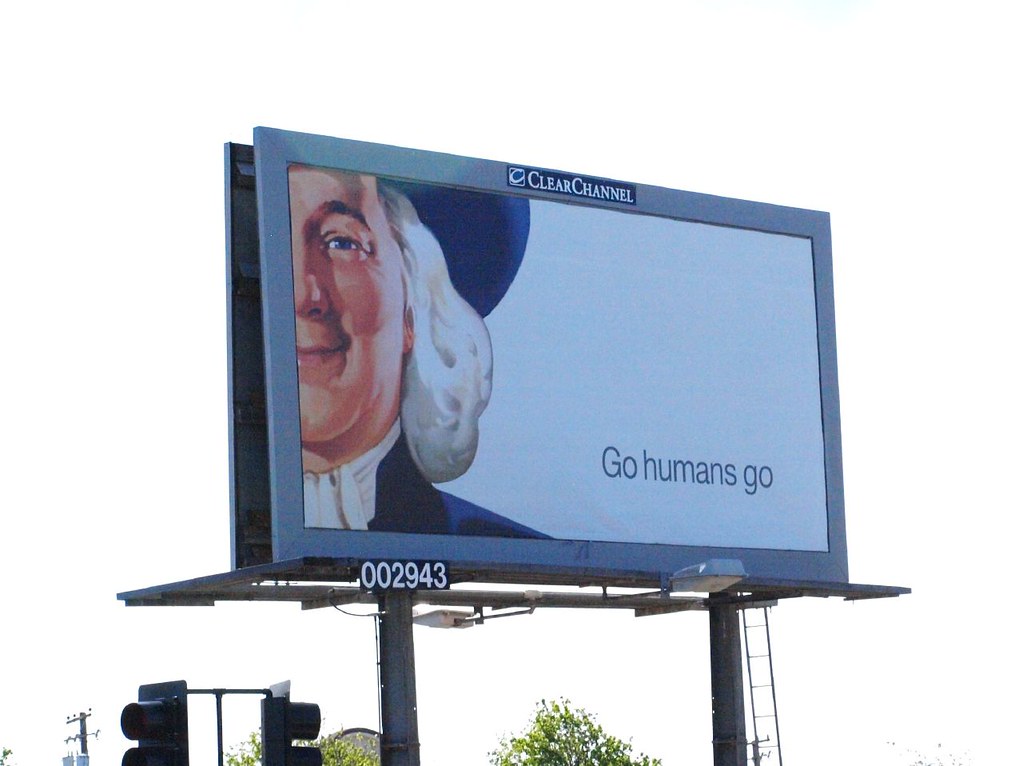This photograph, taken from inside a vehicle, captures a roadside scene featuring a prominent billboard. The billboard, supported by two metal columns anchored at the base with ropes, is elevated by flat metal structures above these columns. It is framed with a silver border displaying the logo "Clear Channel."

At the focal point of the billboard, there is a white background featuring an image of a man with white hair wearing a black hat, white undershirt, and black suit. Beside him, in blue text, the phrase "Go Humans Go" is written, adding a hopeful message to the advertisement.

Below the large billboard, there is a smaller black sign displaying the number "002943." Flanking this sign are two black streetlights, and the scene is further framed by the presence of several trees visible beneath the billboard. The overall setting suggests a tranquil roadside area, providing a backdrop to this striking visual advertisement.